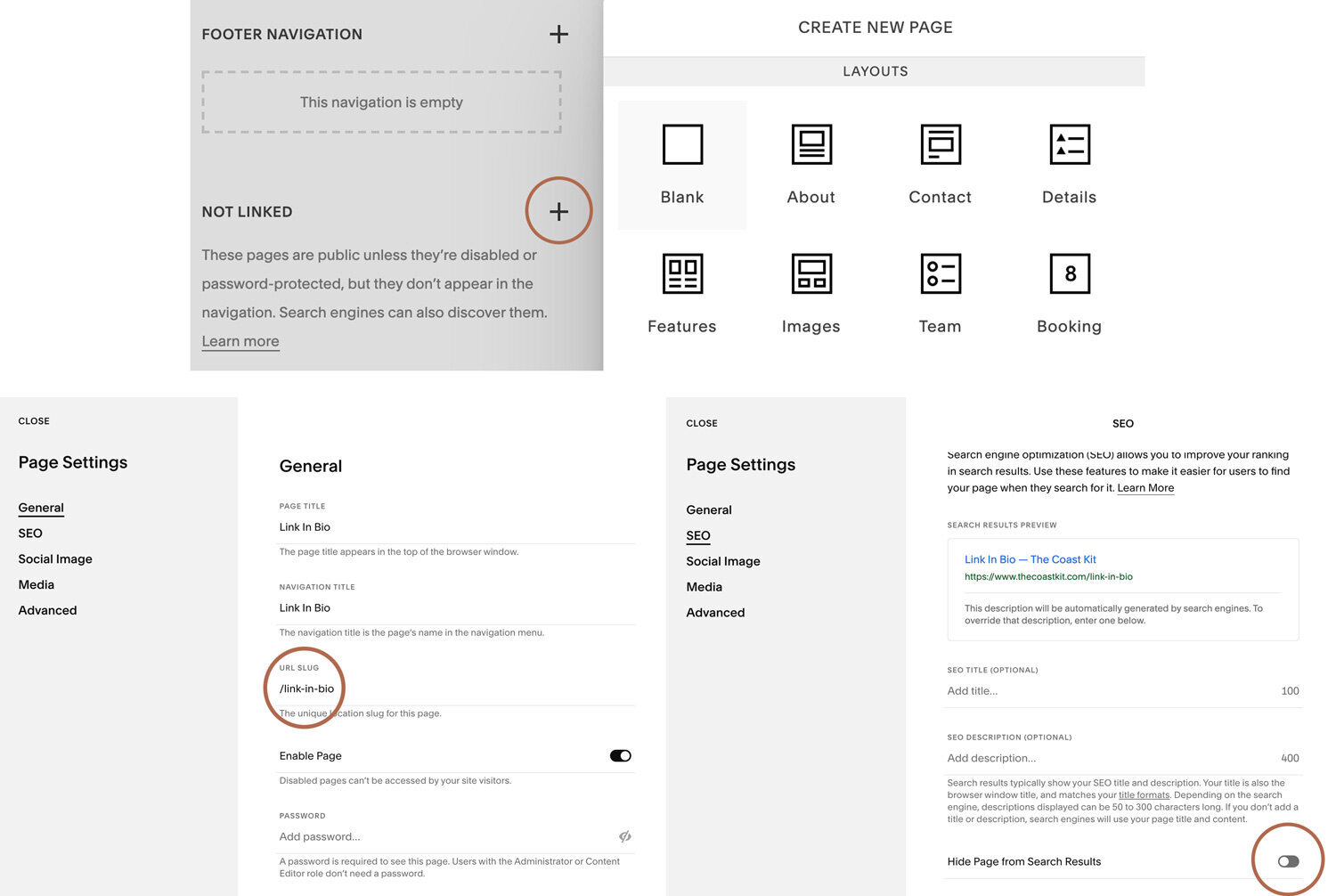Here is a detailed and cleaned-up description for the provided image caption:

---

The image showcases a section of a website, characterized by its white backdrop. On the upper left-hand corner, there is a gray box with black text. The top left-hand corner of this gray box reads "Filter Navigation." Directly beneath this text is a long box outlined by gray dashes, containing the black text "This navigation is empty." Adjacent to the "Filter Navigation" text is a black checkmark. Below the gray box, it states "This navigation is empty." In bold black text, the phrase "Not linked" is displayed on the left-hand side. Beneath this, it explains in smaller black text that "These pages are public unless they are disabled or password-protected, but they don’t appear in the navigation. Search engines can also discover them." Following this is an underlined "Learn more" link.

On the right-hand side of the "Not linked" text, there is a black plus symbol encircled in red. Moving further to the right, outside of the gray box, near the center-top of the page, the text "Create New Page" is displayed. Below this, a gray bar houses the black text "Layouts."

Underneath this gray bar, there are two rows of black icons, each labeled beneath its respective icon. The first row comprises a white box labeled "Blank," a black box with lines and another box inside labeled "About," a white box labeled "Contact," and a black box labeled "Details." The second row features four black boxes labeled "Features," "Images," "Team," and "Booking," respectively. Notably, the "Booking" icon includes a white number eight.

On the bottom left of the image, a gray bar labeled "Page Settings" is visible next to a partially open white page labeled "General." Adjacent to this is a downward-facing gray box labeled "Page Settings," followed by a white box marked "SEO." The SEO section contains several lines of black text that are not entirely legible, forming a vertical row.